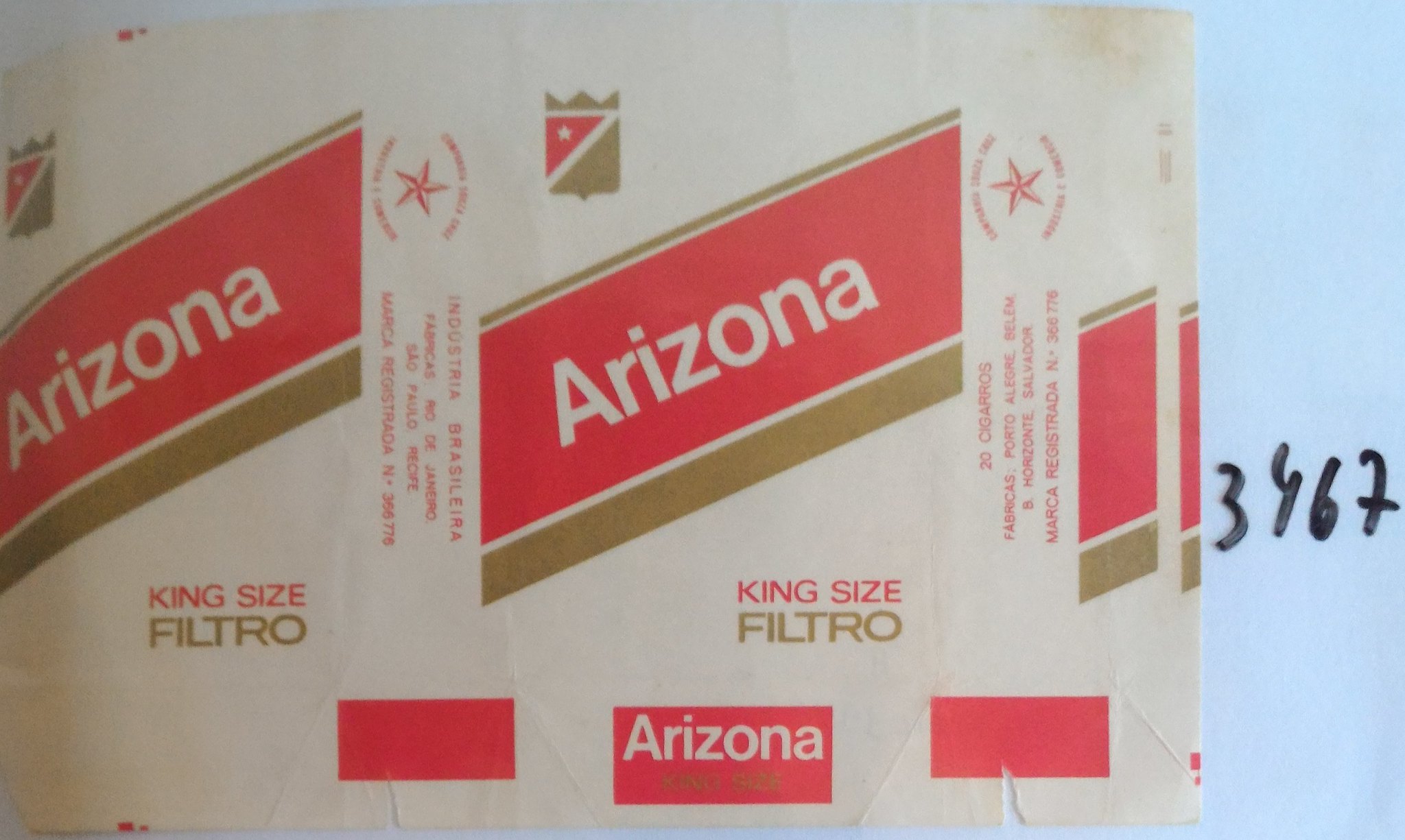The photograph captures a preserved, flattened cigarette packaging, showcased as an artifact in what appears to be a historical archive. The yellowed paper indicates its age, and it bears the number 3467 written in black marker on a light blue background, likely as an exhibit identification. The brand name "Arizona" is prominently displayed in white text on a red diagonal stripe, accompanied by gold detailing. Below the name, "King Size Filtro" is printed, with "King Size" in red and "Filtro" in gold. The packaging features additional text and patterns, and though the wrapper is torn and imperfect with a missing piece in the bottom right corner, it remains an intriguing piece of tobacco memorabilia. The repetitive design and vertical text, possibly in Portuguese reading "industrial brasileira," reinforces its vintage and international character.